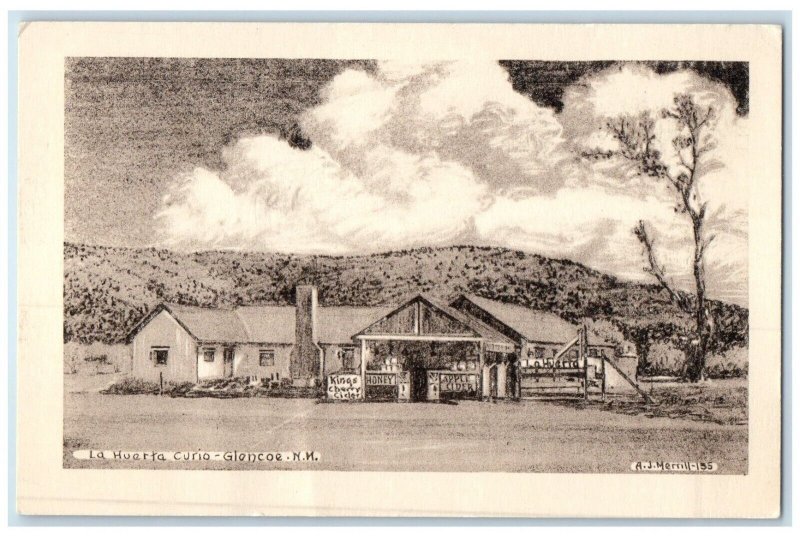The image is a sepia-toned drawing depicting a homestead set in a wide-open field in Glencoe, New Mexico. Centered in the scene is a building, identifiable as a home, which has a chimney at the front. In front of the home, there is a small stand selling honey and apple cider with a sign overhead reading "King's Charter" or possibly "King's Circle." Behind the home, a large hill or mountain rises up, crowned by a vast sky filled with detailed white clouds. To the right-hand side of the image stands a tall, slim tree. On the bottom-left corner of the image, there's an inscription that reads "La Huerta Curio, Glencoe, New Mexico," while the bottom-right corner bears the artist's name, "A.J. Merrill," followed by a partially legible number that appears to be 135. Despite some ambiguity in the finer details, the drawing is well-lit and clearly visible.